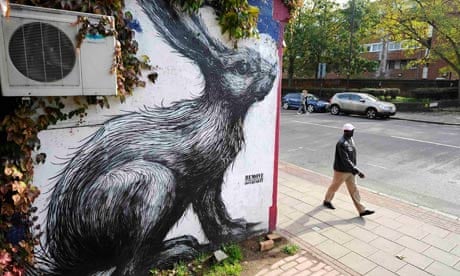This photograph captures an urban scene featuring the side of a white-painted brick building adorned with a large black-and-white mural of a rabbit or hare with long fur. The rabbit, positioned at the corner of the building and facing the street, dominates the wall and appears to be about 12 feet high and 15 feet across. In the upper left corner above the mural, there is a noticeable air conditioning unit with brown vines weaving around it and crawling up the building.

In the foreground, a middle-aged man wearing a white baseball cap, a black shirt, and khaki pants is walking along a brick sidewalk that is adjacent to the building. He is moving from left to right in the image. To his left is a two-lane street with a couple of cars parked along the side. Across the street, we can see additional buildings, trees, and walls partially covered by hedges. The overall setting suggests a modern residential area, possibly up-and-coming, characterized by its mix of urban and natural elements.